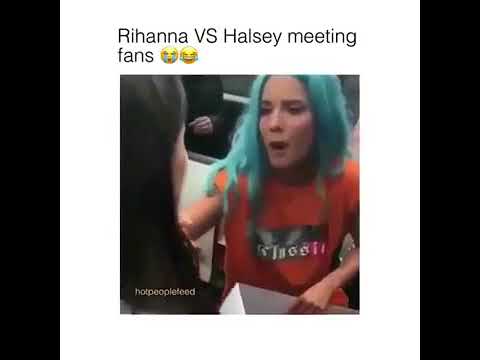In this candid image titled "Rihanna vs Halsey Meeting Fans," a woman with striking turquoise-green hair and a reddish-orange tank top engages in a conversation with another woman whose back is to the camera. The second woman has shoulder-length brown hair. The turquoise-haired woman appears to be holding a rectangular white box. The encounter is captured with the text "Rihanna vs Halsey meeting fans" at the top, accompanied by a crying and laughing emoji. The image is framed by a white border, which is in turn bordered by black, with additional text "hot people feed" displayed in the lower left corner.